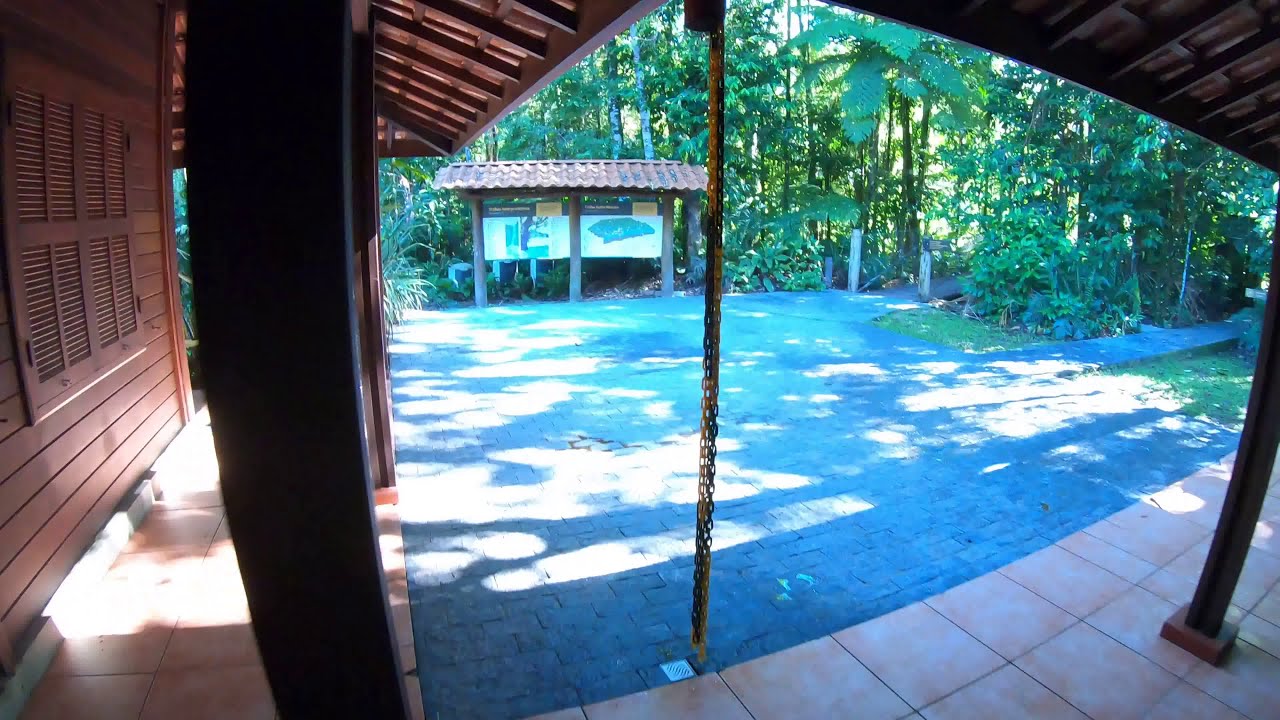This detailed color photograph captures an outdoor scene viewed from underneath the awning of a brown wooden building, which features support beams and a chain hanging from the ceiling down to a brick-paved patio. The photograph appears to be taken from the corner of the building's wrap-around porch, facing out towards a quaint brick plaza surrounded by lush greenery. Dominating the mid-left background is an informational sign with a mini-tiled roof, displaying a map of the rainforest jungle beyond. Multiple walkways, either paved with brick or cement, meander into the dense, leafy vegetation, reinforcing the impression of a park-like or garden setting. The day is sunny, illuminating the tall trees and foliage with vibrant green hues.